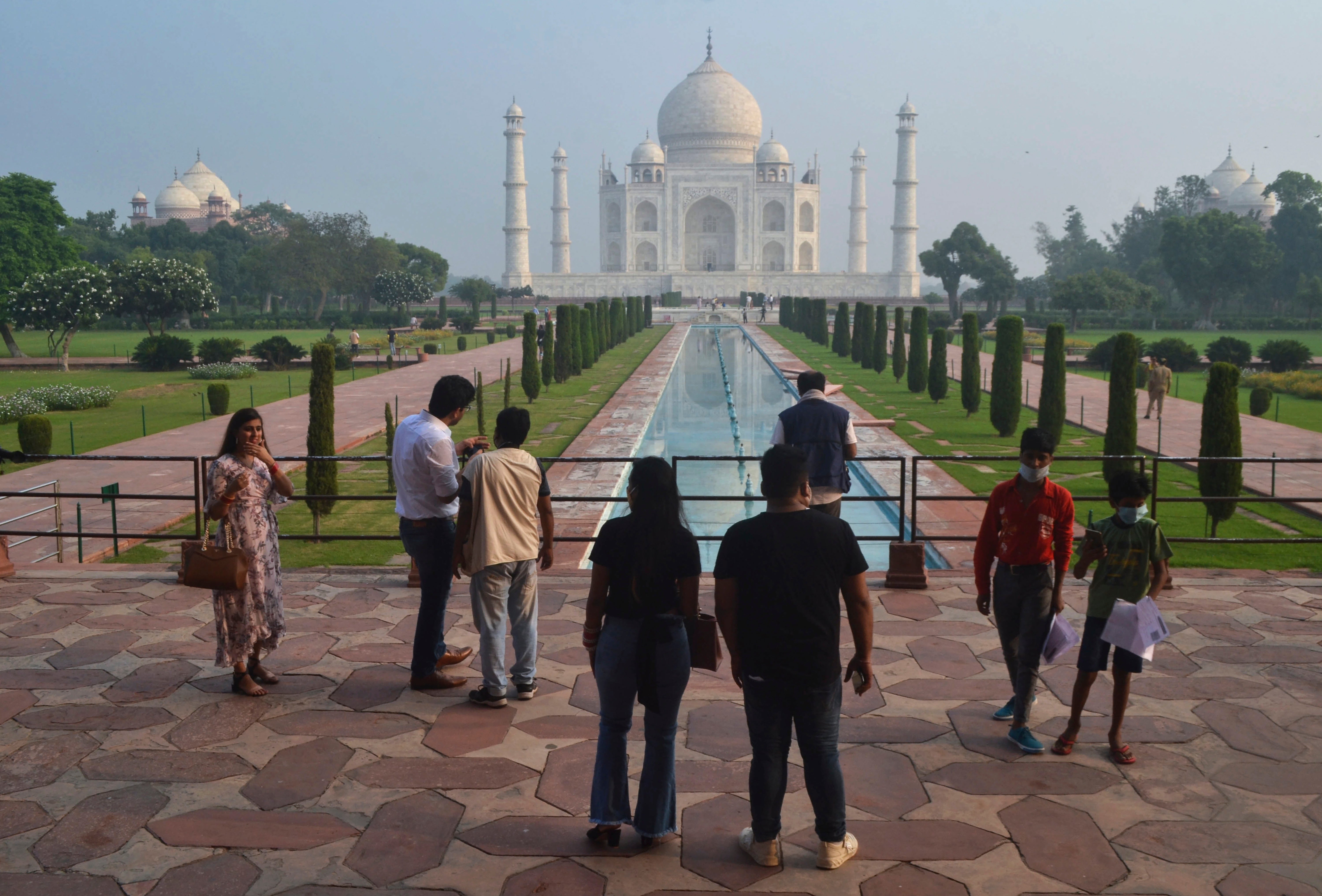The image depicts a scene reminiscent of the Taj Mahal in India, a striking architectural marvel characterized by its pristine white facade. The central structure features an impressive, large white dome surrounded by four intricately carved pillars or posts. Topped with a spire, the building emanates historical grandeur. In the foreground, a long, narrow reflecting pool extends from the base of the structure towards the viewer, flanked by reddish-brown terracotta walkways. This pool and the adjacent paths are lined with lush trees and greenery, contributing to the symmetrical and serene landscape. Visitors, including children and a couple standing prominently in the center, are seen mingling and taking photographs along the stone pathways, capturing the ambiance of this iconic, sunlit yet slightly overcast day. In the distant corners of the image lie additional buildings, partially obscured by the verdant foliage, further emphasizing the grandeur of the setting.